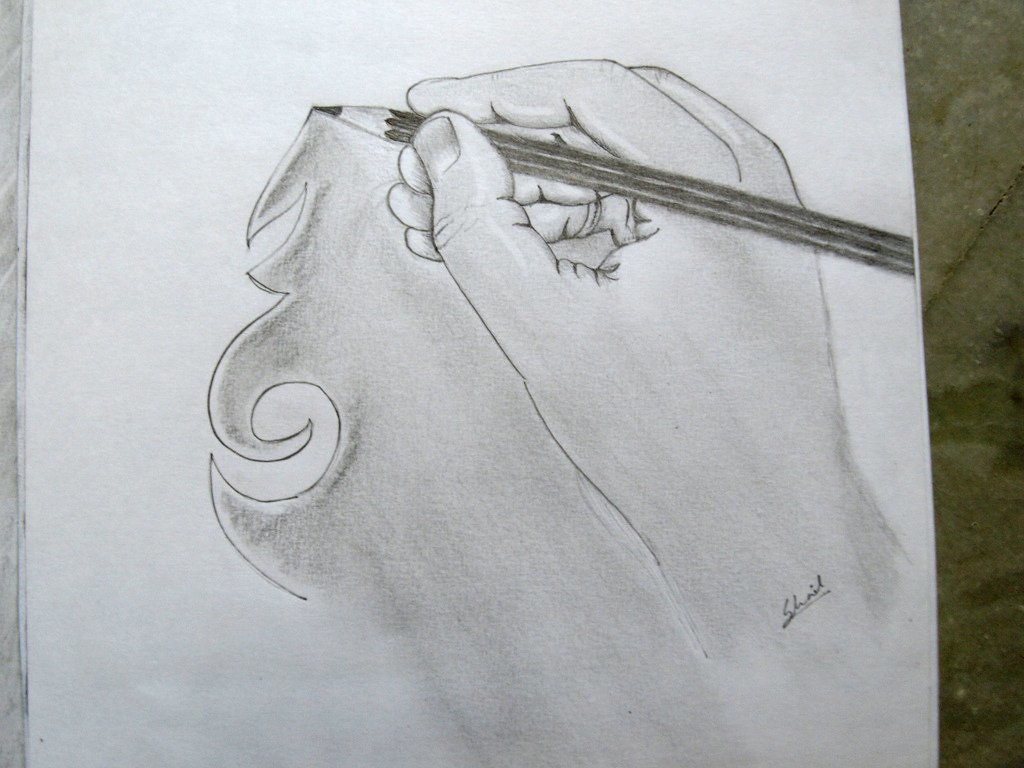The color photograph showcases a detailed pencil sketch on textured white sketchbook paper, placed on a green marble-patterned surface, likely a kitchen countertop. The focal point of the artwork is a realistic depiction of a hand holding a colored pencil, sketching an intricate arrowhead or Celtic tattoo-like design with interwoven curls. The hand is depicted simply, without any jewelry or nail varnish, extending just below the wrist where the artist's scripted signature, "S-H-A-I-D," is visible. The sketched design includes some light shading, adding depth and dimension to the composition.